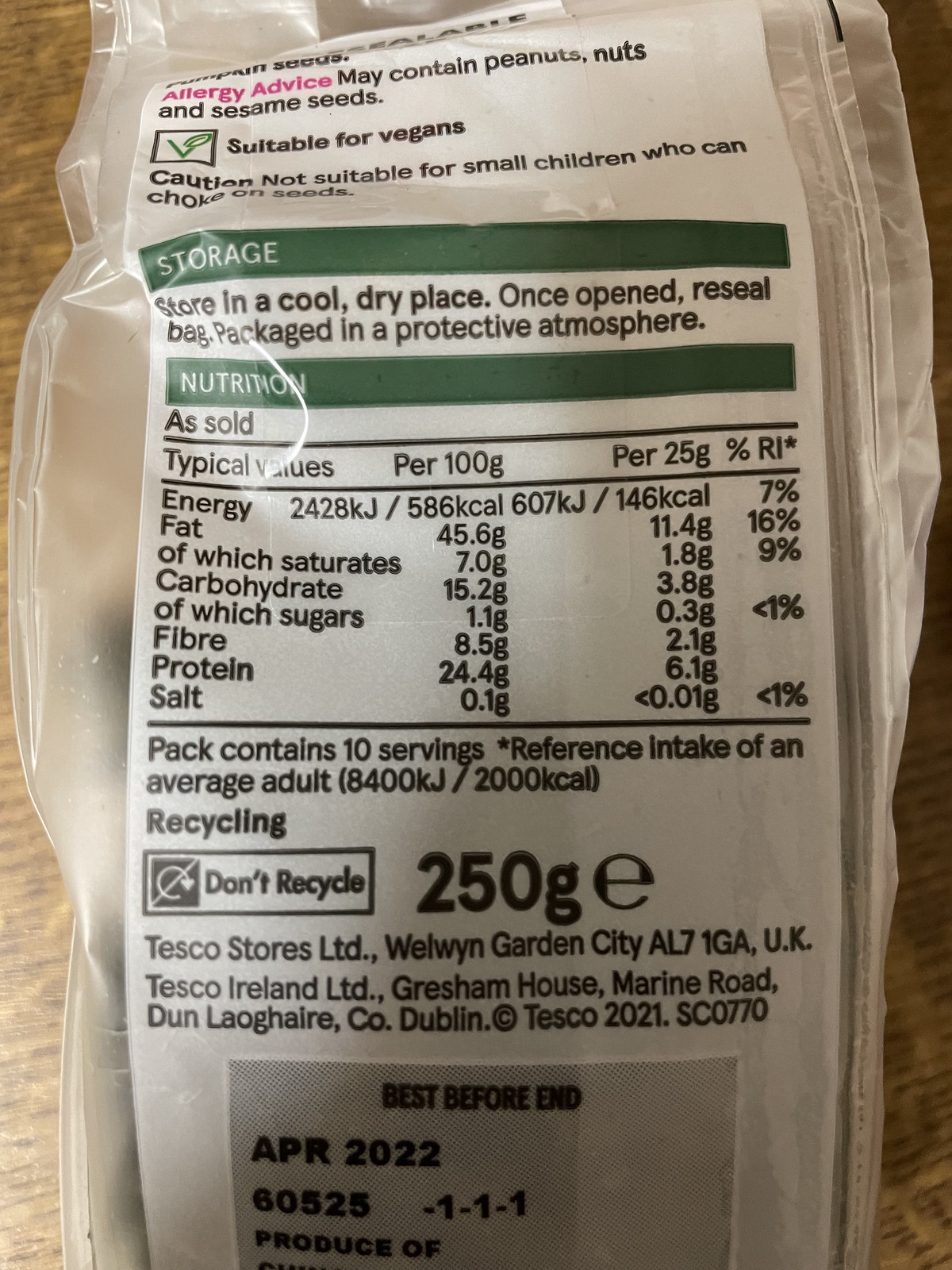The image is of a package's backside, placed on a wooden tabletop, encased in a clear plastic wrapper. This package, suitable for vegans but not for small children due to choking hazards from seeds, provides an allergy warning indicating it may contain peanuts, nuts, and sesame seeds. Detailed storage instructions suggest keeping the item in a cool, dry place and resealing the bag after opening to protect the atmosphere. There is a visible nutrition label highlighting various facts such as a high-energy content and fat levels. The package weighs 250 grams and instructs not to recycle it after use. The product originates from Tesco, with information provided for both Tesco Stores LTD in Welwyn Garden City, UK, and Tesco Ireland LTD in Dublin, including a best before date of April 2022.